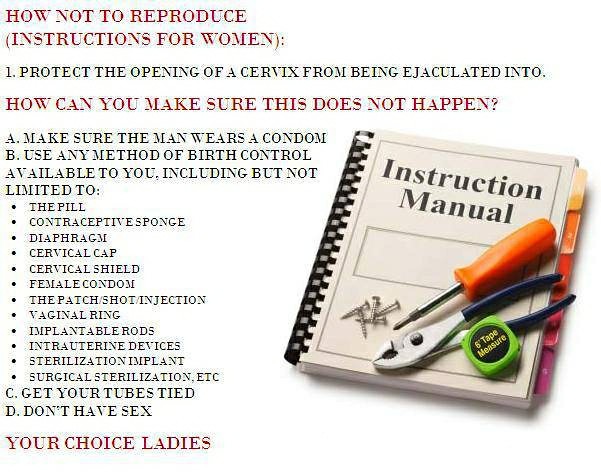The image is a detailed infographic styled as an instruction manual, suitable for inclusion in a PowerPoint slide or social media post. It features a white background with the title "Instruction Manual" in black letters, adorned with visual elements such as an orange-handled Phillips screwdriver, a pair of pliers with dark blue handles, a lime-green tape measure labeled "six foot tape measure" in yellow letters, and various screws. To the left, there's a red heading that reads "How Not to Reproduce" with the subtitle "Instructions for Women" also in red. Below this, in black letters, it advises, "Protect the opening of the cervix from being ejaculated into" and lists several birth control methods: "Make sure the man wears a condom," "Use any method of birth control available to you," including the pill, contraceptive sponge, diaphragm, cervical cap, cervical shield, female condom, patch, shot/injection, vaginal ring, implantable rods, intrauterine devices, sterilization implant, or "Get your tubes tied." It concludes with "Don't have sex." At the bottom, in red letters, it emphasizes: "Your choice, ladies."